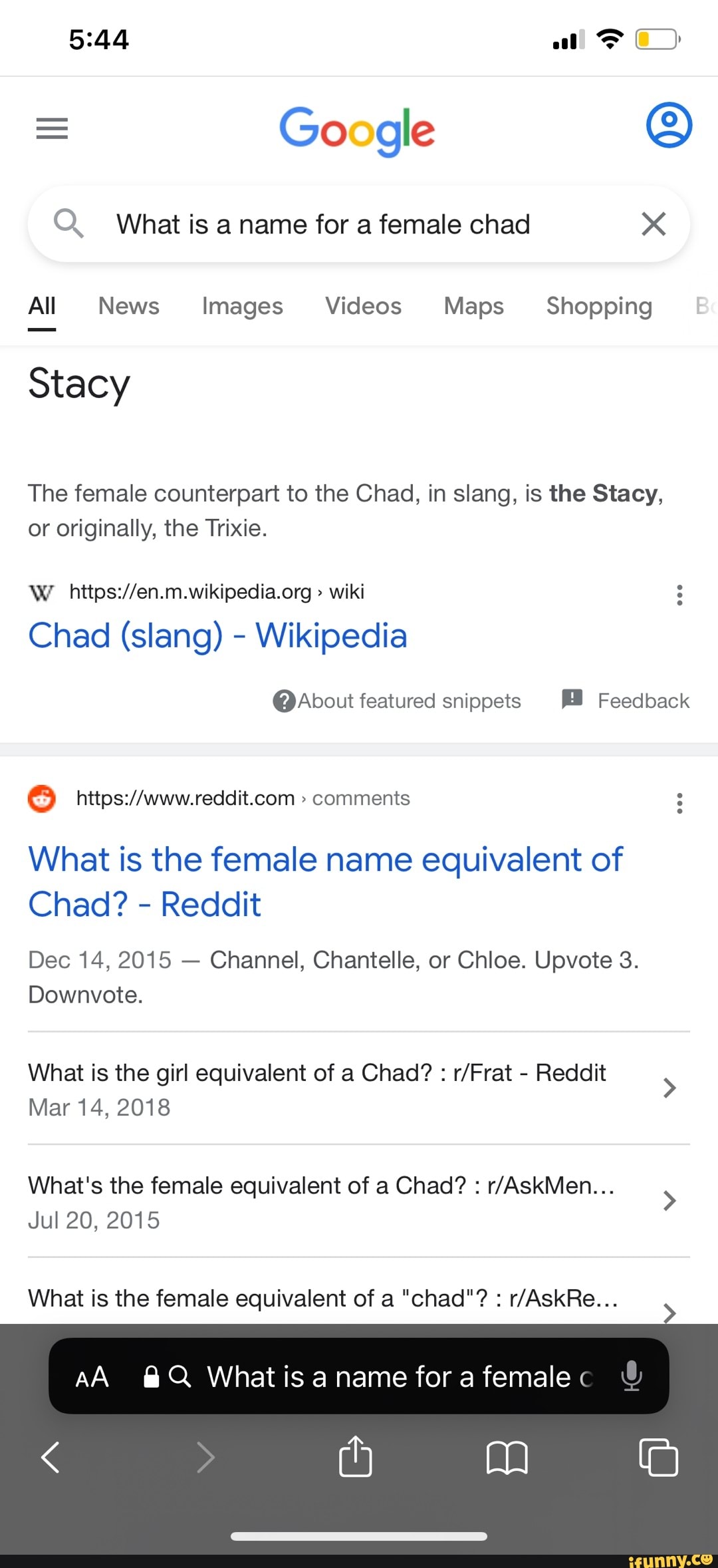The image features a search query about the female equivalent of the term "Chad," commonly used in internet slang. The screen displays multiple search results and forum discussions from various platforms, including Reddit and Wikipedia, with users suggesting names like "Stacey," "Trixie," "Chanel," "Chantel," and "Khloe." The search bar prominently displays the question, "What is a name for a female?" Above the search bar, navigation icons such as back and forward arrows, along with upload and bookmark options, are visible. The image also shows interface details like a white line at the bottom with the website watermark "ifunny.co" on the bottom right. The top right corner features a yellow battery symbol and Wi-Fi data indicator, while the top left corner shows the current time as 5:44.